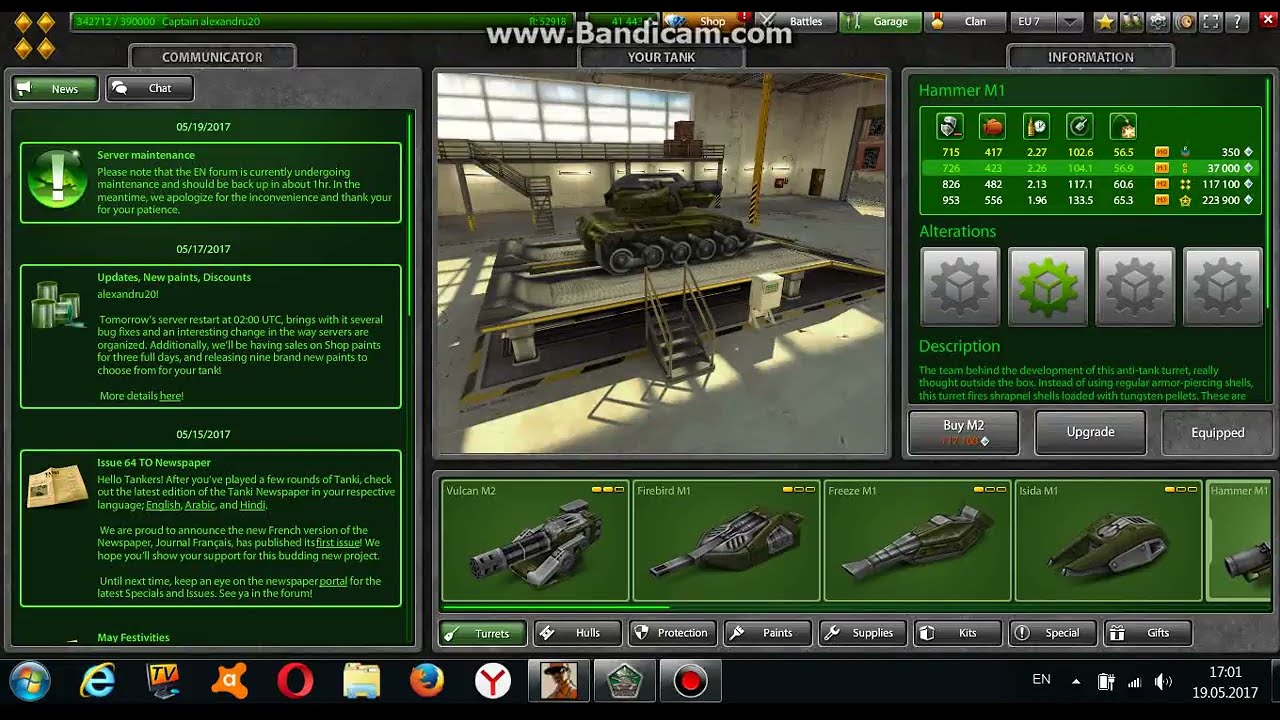The screenshot displays a video game customization screen, most likely for a tank game, set inside a large concrete warehouse with big windows at the top. In the center of the image, a green military tank is positioned on a metal platform. Surrounding the tank are various customization options: directly below it are selectable weapon options such as Vulcan M2, Firebird M1, and Freeze M1; on the upper right side, there is another panel showing the Hammer M1 and detailed stats about the tank. On the left side of the screen, a green panel with light green text serves as a data log, listing communications and chapter completions with dates. The background has a dark green hue, contrasted by the light green text. At the very bottom of the image is a Windows taskbar displaying icons like the Windows logo, Internet Explorer, Opera browser, Firefox, and others, including time, date, and volume control in the lower right corner.